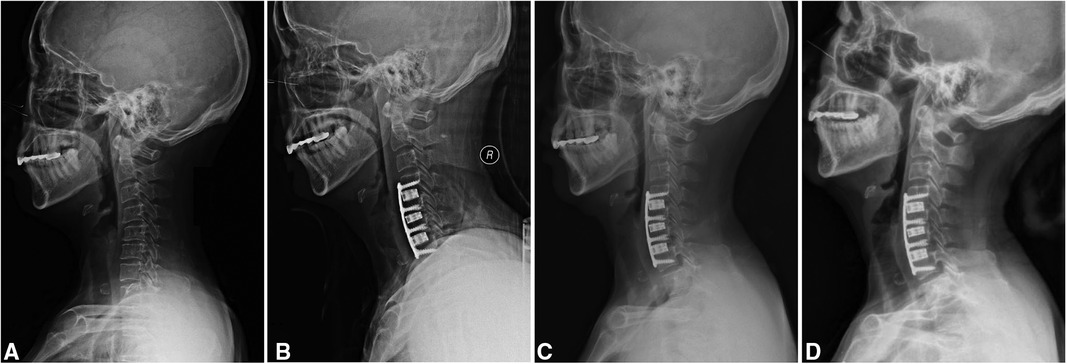The image consists of four sequential black-and-white x-ray scans of a person's neck, labeled A, B, C, and D from left to right. Each x-ray shows a side view of the person's head, neck, and upper shoulders. Scan A appears to be a standard x-ray showing the person looking straight to the left without any significant highlights or markings. In scan B, the individual’s head tilts slightly forward, and three distinct markers or additions are noticeable in the neck area, indicating an area of interest or medical intervention. Scan C shows the person looking straight again with the three additions still present in the neck, maintaining the same orientation as in the first scan. Finally, in scan D, the individual's head is seen leaning back slightly, with a noticeable curve in the spine or neck area. These images seem to track the progression or treatment of a condition in the neck, perhaps used for educational or diagnostic purposes in a medical context.